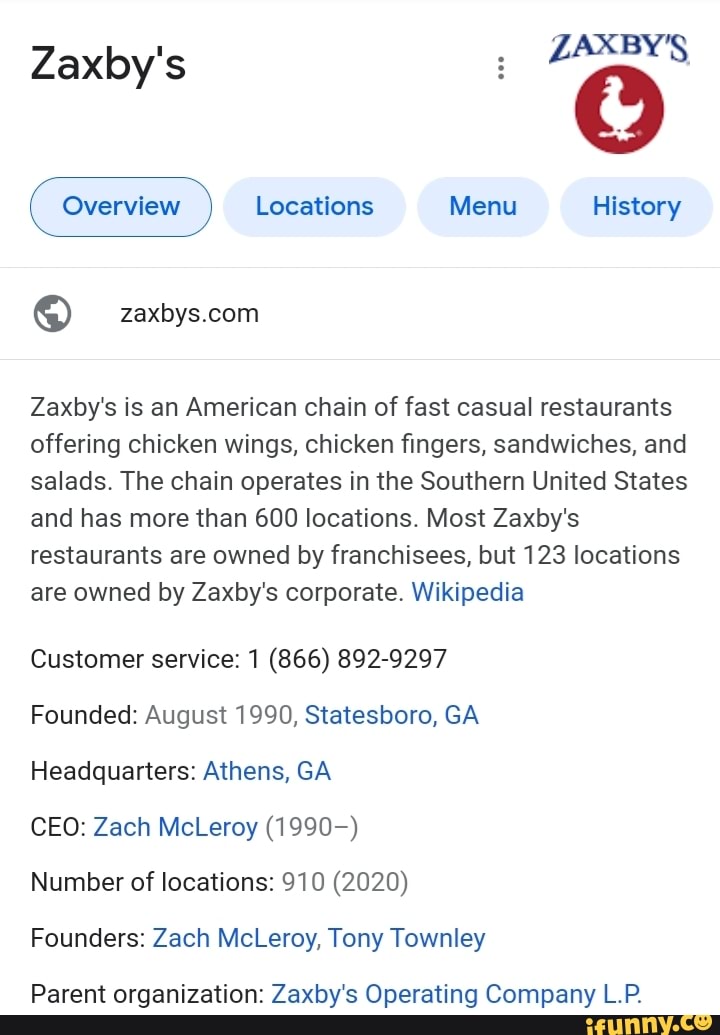Screenshot Details:
- Source: Google Maps 
- Content Type: Cropped screenshot displaying specific information about a place

Description:
The image is a cropped screenshot taken from Google's map function, specifically showcasing details about the fast-casual restaurant chain, Zaxby's. On the right-hand side of the screenshot is a prominent icon: a red circle featuring a white silhouette of a chicken, with the word "Zaxby's" written in blue text above it.

Navigation Options:
- The screenshot features four hyperlinked, selectable buttons labeled:
  - Overview (selected)
  - Locations
  - Menu
  - History

Overview Tab Details:
- A web link to Zaxby's official site: Zaxbys.com
- A concise Wikipedia blurb describing Zaxby's as an American chain offering chicken wings, chicken fingers, sandwiches, and salads.

Additional Information:
- The Overview tab also provides detailed information, including:
  - Headquarters location
  - CEO's name
  - Number of locations
  - Year of establishment
  - Customer service contact number